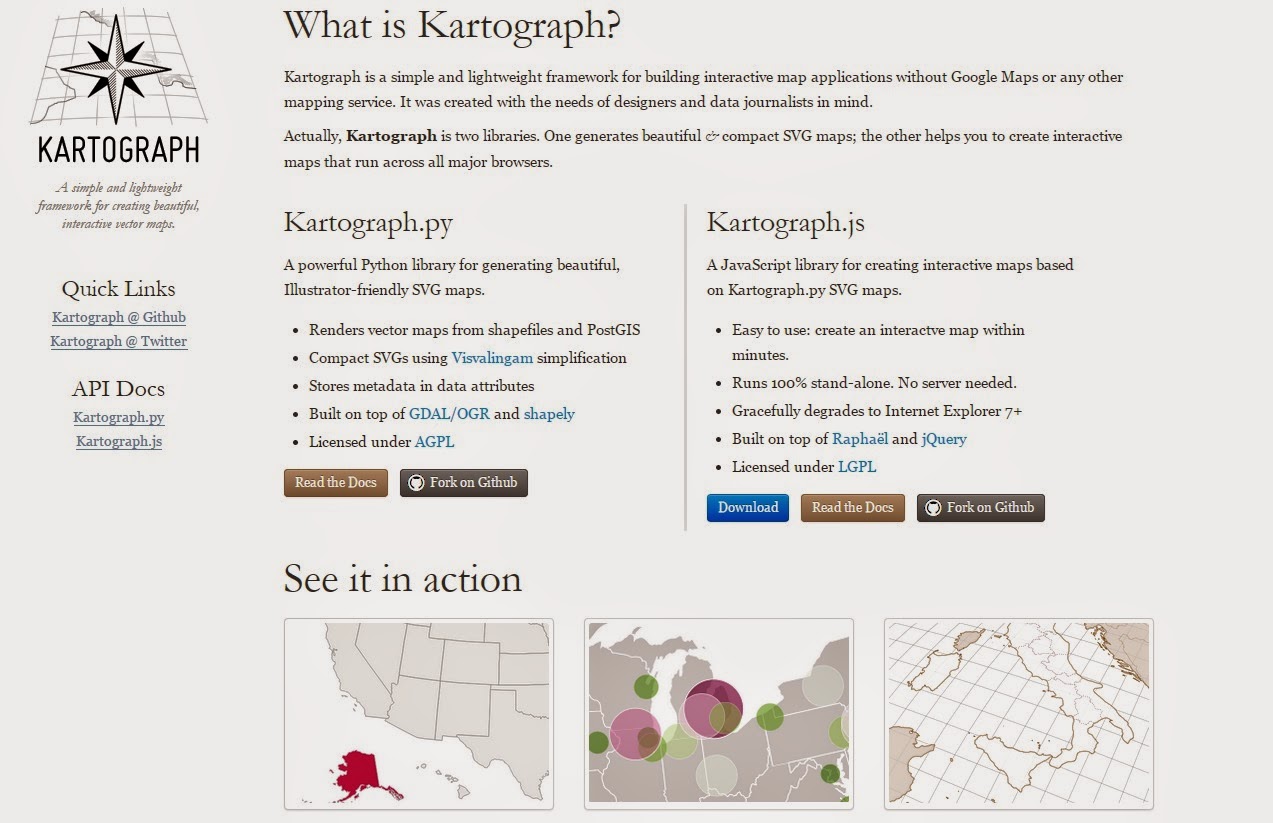The image depicts a web page with a light pastel gray background. In the upper left corner, there is an eight-pointed star situated on a 3D-looking grid composed of horizontal and vertical lines, forming a square pattern. Below the star, the word "Cartograph" is written in black text. To the right of the star, in black text, the phrase "What is Cartograph" is displayed. Beneath that, in smaller print, a description reads: "Cartograph is a simple and lightweight framework for building interactive map applications." Additional definitions of Cartograph are provided further down. At the bottom of the image, there are three smaller images of maps and cartographs. From left to right, they depict: 1) A cartograph of the United States highlighting the West Coast and the state of Texas; 2) A series of maps with purple and green circles; and 3) Another unspecified map-based illustration.